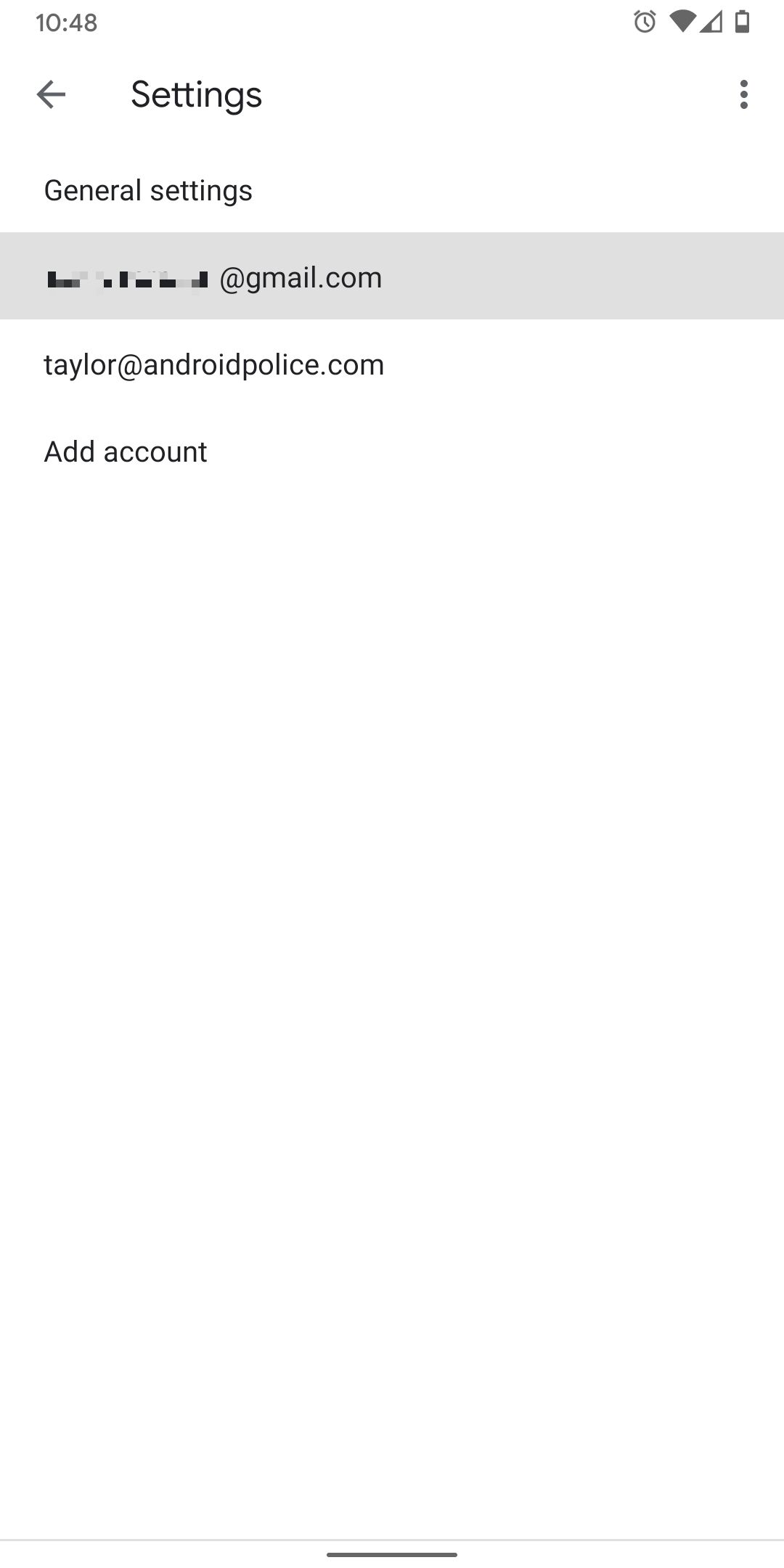This image, captured from the screen of a smartphone, displays various interface elements typical of a settings menu. At the top right of the screen, the time is shown as "10:48," next to indicators for Wi-Fi connectivity and signal strength. Below these icons is a battery symbol, revealing that the device's battery life is roughly one-third full. 

Centered at the top, an arrow icon pointing to the left is positioned next to the word "Settings." On the right side, three vertical gray dots indicate a menu. Beneath this header, in slightly grayish print, the text "General settings" is displayed. Below it, several blocks are used to obscure a personal email address, which ends with "@gmail.com."

Further down, another email address, "Taylor@androidpolice.com," is clearly visible, followed by an "Add account" option. The main portion of the screen is stark white, providing a clean backdrop. At the very bottom, a faint gray line stretches across the width of the display, with a shorter, darker gray line placed in the center.